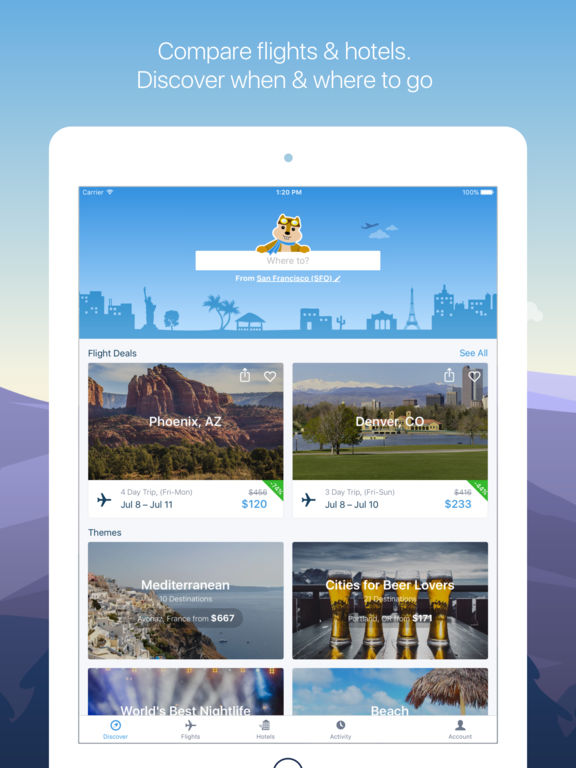The image features an elegant gradient background that transitions from a light blue at the top, down to a light purple, and eventually into a darker purple before melding into white in the middle. At the upper-middle section, bold text reads "Compare Flights and Hotels. Discover when and where to go."

Central to the image is a graphic representation of an iPhone, displaying a few specific elements: at the top left, "Carrier" is written in blue, while the top right shows a battery at 100% and the time is displayed as 1:20 PM in the center.

Beneath this, a white rectangular search box contains the prompt "Where to?" Underneath, it specifies a starting point: "From San Francisco (SFO)." Additional options are laid out with "Flight Deals" on the left and "See All" on the right.

A series of six enticing destination images occupy the lower section of the iPhone screen:

1. **Phoenix, Arizona**: Illustrated with desert scenery, labeled for a four-day trip from Friday to Monday, July 8th through July 11th. The price is $120, significantly reduced from $456.
   
2. **Denver, Colorado**: Shown for a three-day trip from Friday to Sunday, July 8th through July 10th with a price tag of $233.
   
3. **Mediterranean**: Highlighting 10 destinations starting from $667.
   
4. **Portland, Oregon**: Themed for beer enthusiasts, starting from $171.
   
5. **World's Best Nightlife**: Partially visible below.

6. "Beach or Other Categories": Along the bottom edge, suggesting further options.